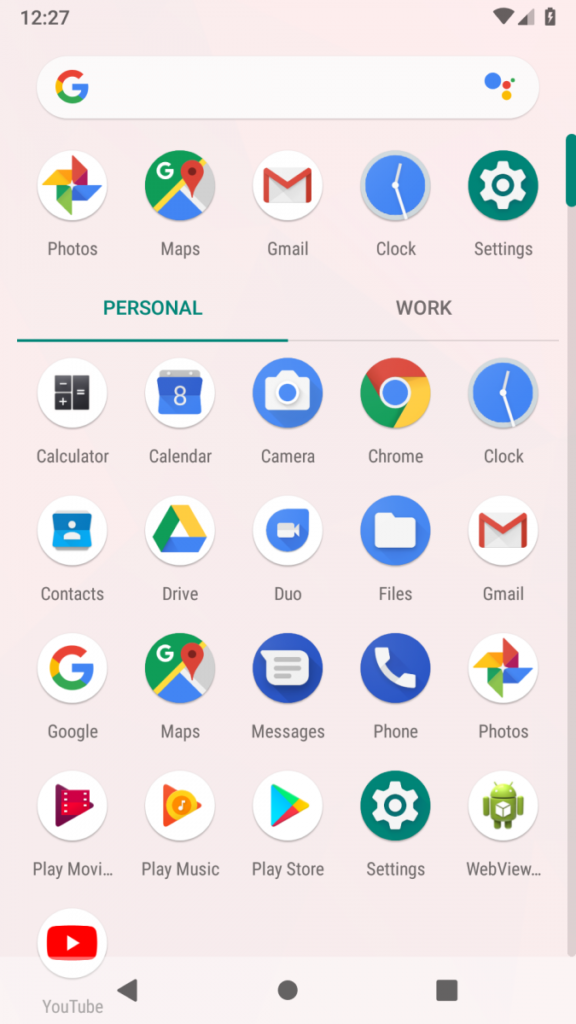This is a detailed color image, seemingly a screenshot from a mobile device, possibly a phone or a tablet with mobile connectivity. The upper right-hand corner displays a Wi-Fi icon, signal strength indicator, and battery status, while the upper left-hand corner shows the time "12:27." The background is beige, with a Google search bar prominently positioned at the top, featuring the iconic "G" on the left side.

Beneath the search bar is a row of app icons, set against an interface clearly delineated by two tabs labeled "Personal" and "Work," with the "Personal" tab highlighted in green. The right-hand edge of the screen showcases a scrolling indicator with a small green section visible.

Moving downward, there are five rows of app icons. The array includes:
- Calculator
- Calendar
- Camera
- Chrome
- Clock
- Contacts
- Drive
- Duo
- Files
- Gmail
- Google Maps
- Messages
- Phone
- Photos
- Play Movies
- Play Music
- Play Store
- Settings
- Web View
- YouTube

At the bottom of the screen rests a lighter, creamy navigation bar with three distinctive black icons: a triangle for "Back" on the left, a circular "Home" button in the center, and a square for "Recent Apps" on the right. This layout is characteristic of an Android device, although the unique feature of organizing apps into "Personal" and "Work" tabs may indicate a newer Android version or a specific customization.

Despite the detailed visual clues, it's uncertain if this is a standard home screen due to the unfamiliar tab feature, which might be an update beyond older Android versions.